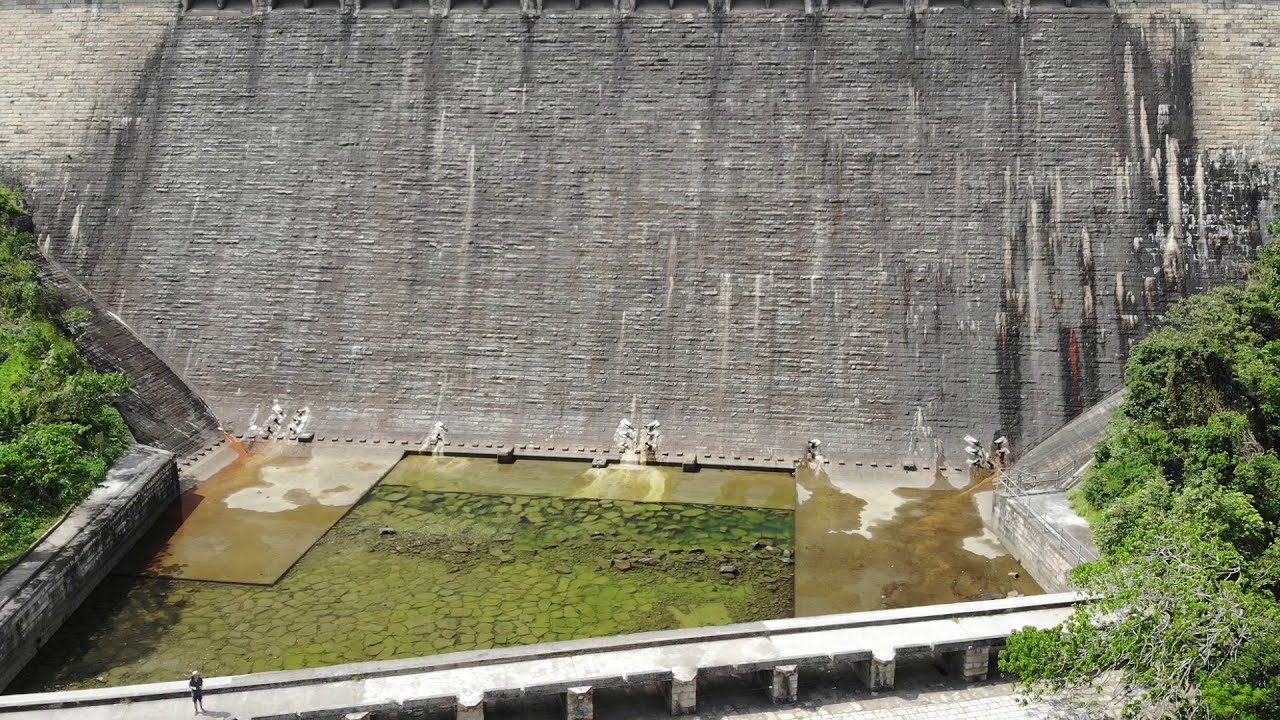The image depicts a large man-made dam with a distinctive slanted, concrete structure that appears to be about 100 to 200 feet tall. The dam is visibly weathered and adorned with white streaks and patches of algae, giving it a worn-out look. This immense structure dwarfs a person standing on a walkway that extends in front of the dam. The individual, dressed in a long-sleeved blue top, capri pants, and a white hat, appears tiny against the expansive backdrop. Below the dam is a shallow, greenish-yellow river, surrounded by levee-like walls with adjoining trees on either side. The riverbed and the water show signs of stagnation and algae growth. Additionally, the left side of the image features a stairway likely used by workers, leading down to the walkway that offers a vantage point of the dam's impressive yet weather-beaten form.